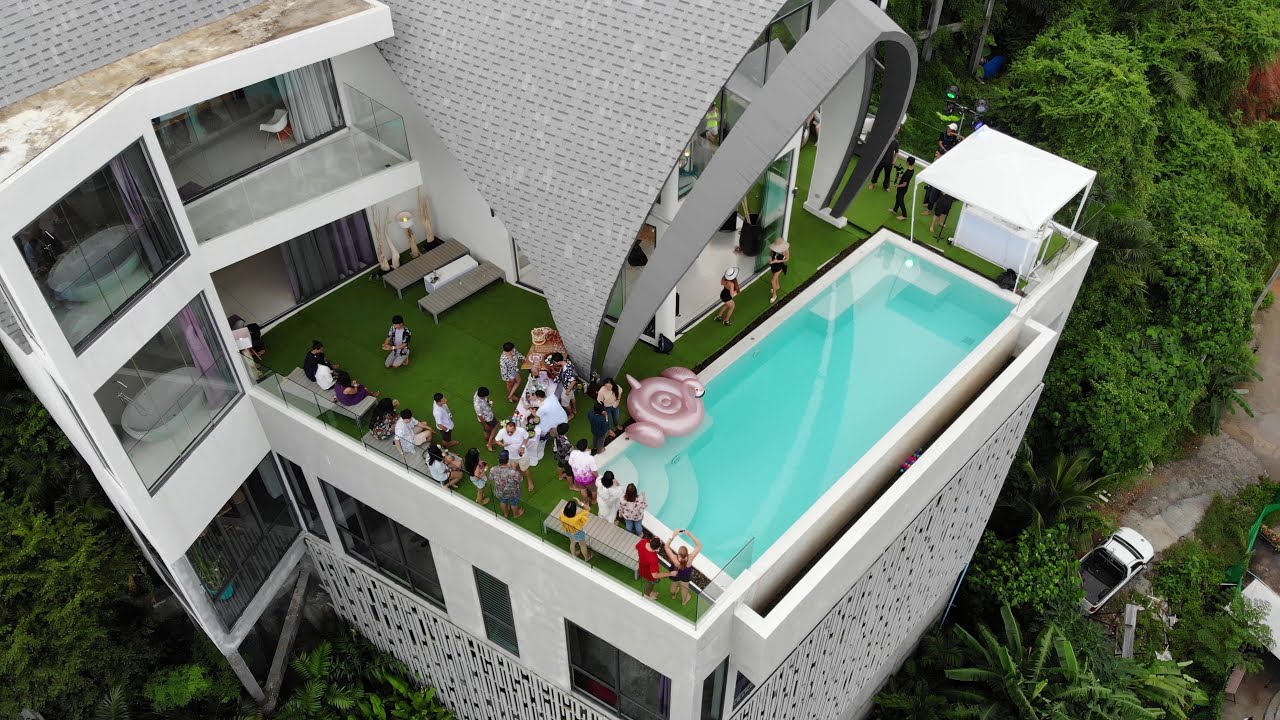This aerial photograph captures the top of a modern, multi-story building, possibly a hotel or high-end apartment complex. The building, characterized by its white tiled exterior and large windows, displays a distinctly modern design with a curved, arch-like gray roof, constructed from what appears to be stone or metal. Dominating the rooftop is a large, rectangular, light blue swimming pool, bordered by green astroturf that provides a lush, grassy appearance.

The scene on the rooftop is lively, indicating a social gathering or party. Numerous people, dressed in casual, colorful attire, are dispersed around the rooftop, engaging in various activities such as chatting, taking photos, and enjoying food from a long white table filled with refreshments. An inflatable swan and a pink flamingo floatie add a playful touch to the poolside environment.

The building stands in what looks like a tropical area, evidenced by the presence of palm trees, grass, and other dense brush near a car park visible at the edge of the image. Additional details include large, possibly luxurious bathtubs that can be seen through some of the windows below the rooftop, enhancing the building's modern and upscale appearance. The overall impression is that of a chic, contemporary space buzzing with social activity.